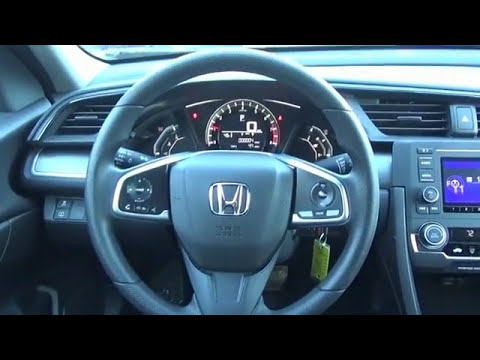The photograph captures the interior view of a Honda vehicle, with the steering wheel prominently centered. Dominating the wheel is the metallic silver "H" emblem of Honda, encased in a rounded square. The wheel is straight, resting on the dashboard that features a lit tachometer and speedometer, indicating the car is in park with a "P." Flanking the steering wheel are various controls, with round buttons on either side and a V-shaped center spoke integrating additional buttons and controls. A laminated yellow keychain dangles from the ignition. On the right side of the wheel, there is a digital display screen for the radio, while the air conditioning controls are on the left. Above the steering wheel, precise gauges inform the driver of speed, mileage, and essential vehicle metrics. Visible through the windshield is a slice of the well-lit interior and part of the car door on the left. The overall interior showcases a sleek, metallic gray design with accents suggesting a high-quality finish. The dashboard also features three foreign characters, possibly in Chinese or Japanese, providing a hint of the car's origin.